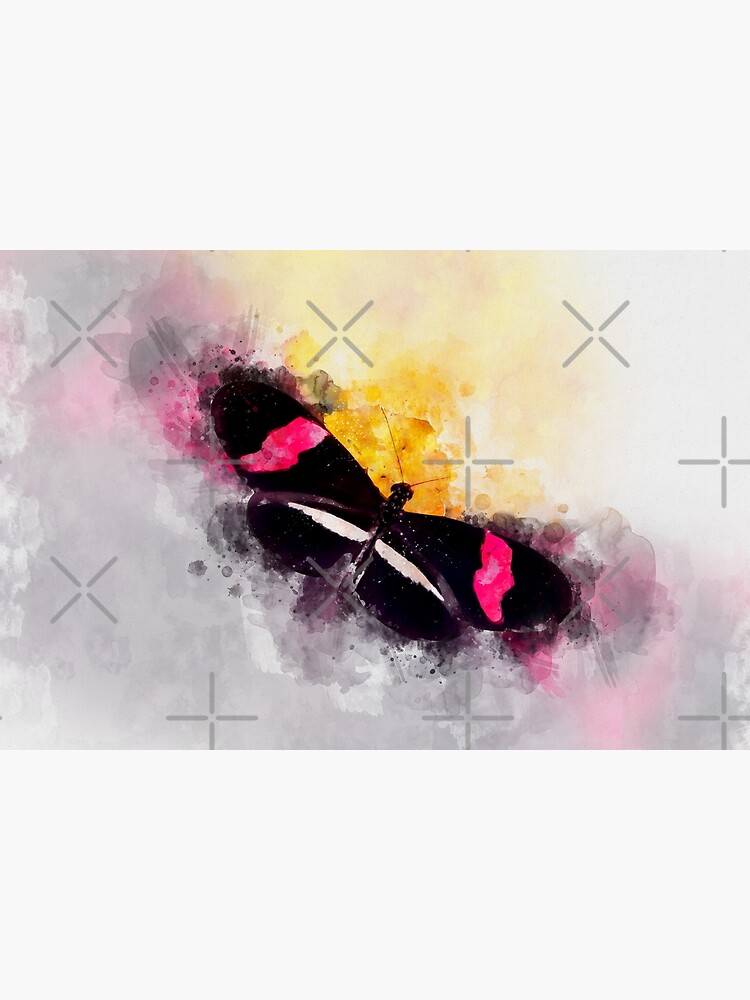This image depicts a modernist-style watercolor painting of a black butterfly or moth, centered horizontally. The butterfly features four wings—two larger front wings and two smaller back wings—and is distinguished by vibrant hot pink stripes along the edges of its front wings. The rear wings display a horizontal pink stripe that spans from one wing to the other. Adding further detail, white stripes cross the tops of these back wings. Black antennas extend from the butterfly's head. Surrounding the butterfly, there are watercolor splotches: bright yellow in front of its head, bright pink behind its wings, and interspersed patches of bright pink and gray behind its back wings. The background transitions from a light gray in the lower left-hand corner to a pale yellow in the upper right-hand corner. Additionally, there are semi-transparent, dark gray X's and plus signs of varying shapes and sizes scattered across the background, imparting a confetti-like effect. The image evokes the sense of viewing the butterfly through a hazy lens, with the colors and forms of the background becoming more diffused and blurred in contrast to the clearer, more vivid depiction of the butterfly in the center.